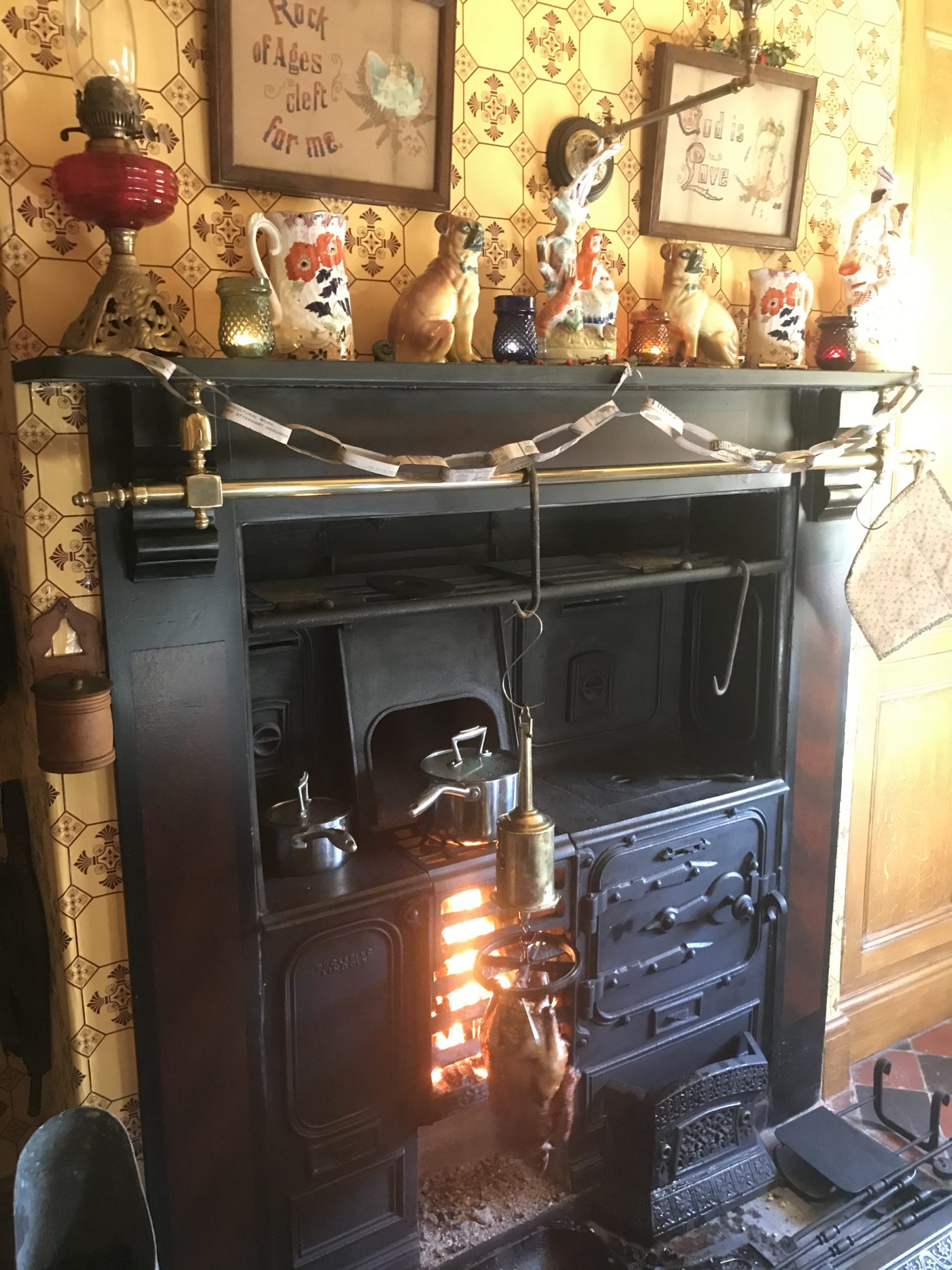The photograph captures a detailed scene of a vintage 1800s iron stove, almost black in color and set into a wall like a fireplace mantle. The stove is lit, with visible flames behind slats near the bottom, where items necessary for its operation are scattered. A notable feature is a spit with a chicken roasting in front of the fire, suspended by a wire from the stove's top. On the stove’s top level, a silver pot sits on a flame, accompanied by a smaller round pot to its left, both with rectangular handles on their lids. Above the stove is a mantelpiece adorned with various knickknacks: ceramic dogs, jugs, old oil lamps, and candles in glass jars. A gold horizontal bar runs across the stove’s upper front. The surrounding wall is decorated with beige tiles featuring diamond and cross patterns. Framed pictures hang above the stove; one reads "Rock of Ages, cleft for me," and another says, "God is love," both in brown wooden frames. To the stove's right is a brown wall section and possibly a door. The floor partially visible below the stove shows a black and brown triangular checkered pattern.